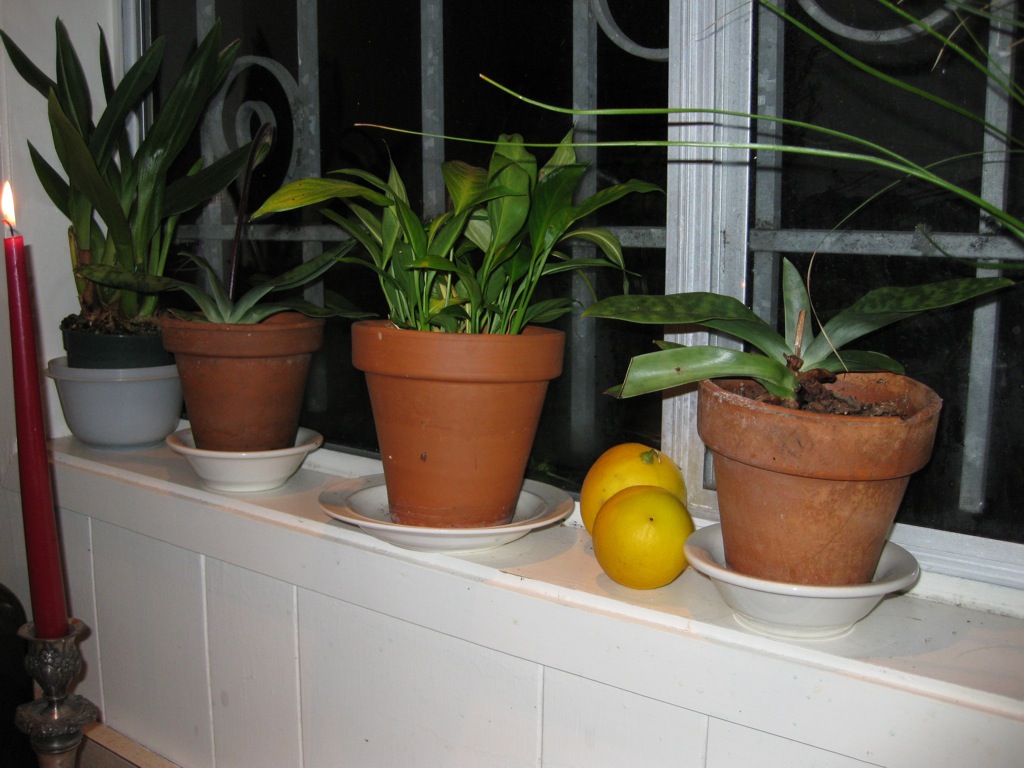This photograph captures a white wooden windowsill adorned with four potted plants positioned against a backdrop of grey-barred windows, hinting at the dark night outside. On the far left, a red lit candle in a decorative dark metal stand softly illuminates the scene. Each plant is housed in a distinct pot; the first plant, in a clay pot, is accompanied by two pale oranges. The second and third plants are also in similar terracotta pots, sporting dark green leaves that reach upwards. The fourth plant, slightly obscured and darker in color, is set in a blue pot, also sprouting tall green foliage. The windowsill, outlined in white wood, supports the pots on white bowls, creating a harmonious yet varied display. The detailed interplay of light, earthy textures, and verdant greens against the sleek metal bars of the window makes for a serene and visually engaging image.